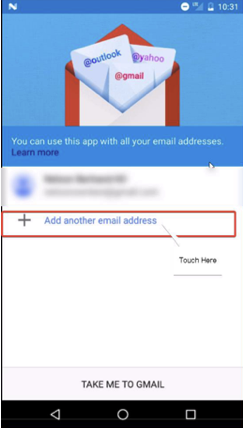This image, captured from a smartphone, depicts a detailed screen interface. At the top, a blue banner features a white letter "N" in the left-hand corner, accompanied by various icons on the upper right, including a small white circle, signal strength bars, a low battery symbol (indicating approximately 20% remaining), and the current time displaying as 10:31.

Below the banner, there's a blue rectangular background highlighting an illustration of a cartoon envelope with red trim in the foreground. The envelope contains three distinct cards. The card in front is white, adorned with the word "Outlook" in blue text. Behind it, another card features "@Gmail" written in red, and the third card displays "@Yahoo" in a pink-lavender font.

Beneath this visual, a darker blue rectangle contains light blue text stating, "You can use this app with all your email addresses," followed by "Learn more" in a slightly darker blue font.

The lower portion of the screen displays a white background with a blurred-out name and icon near the top. Following this, a prominent red rectangle features a blue plus sign and the words, "Add another email address." Adjacent to this, a rectangle with a pointer directs attention to the end of the word "address."

Continuing downward, a pink rectangle contains the phrase "Take me to Gmail" in black font. Finally, the bottom of the screen houses a black banner showcasing three white navigation icons typical to a cellphone interface.